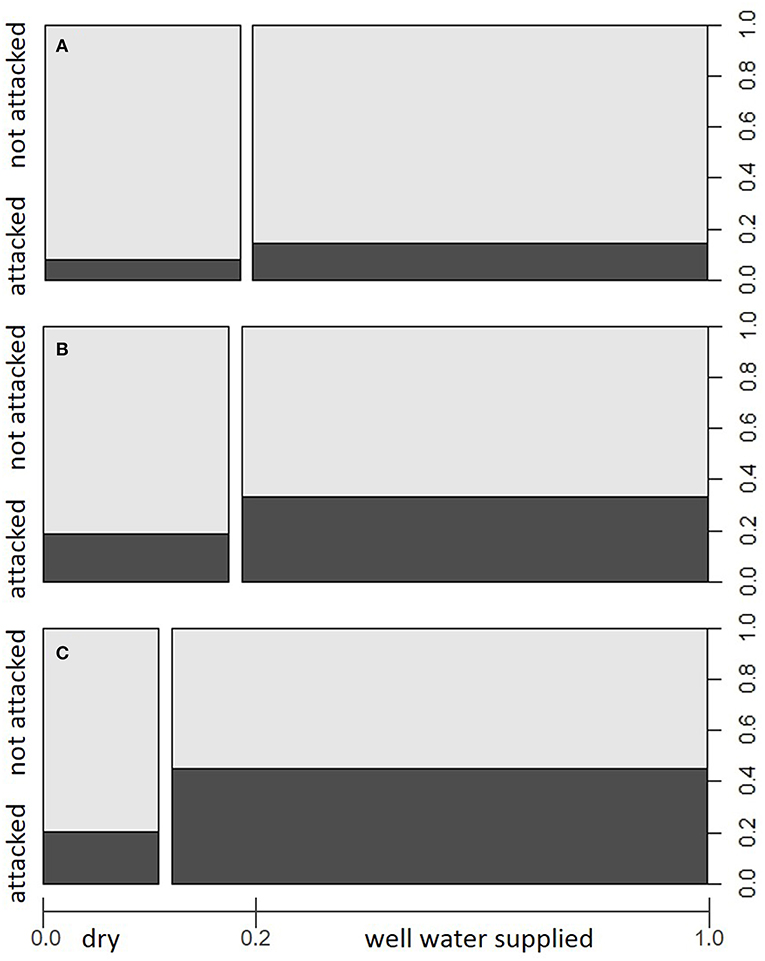The image consists of three vertically stacked bar charts labeled A, B, and C. Each bar chart depicts two sections: one labeled "Attacked" and the other "Not Attacked". The charts use a grayscale to differentiate between these sections, with darker gray representing the "Attacked" condition.

- **Box A**: At the top, the "Attacked" section is represented by a dark gray line spanning from 0 to approximately 0.2 on a horizontal scale ranging from 0 to 1.0. The section labeled "Not Attacked," represented by a lighter gray, lies above the "Attacked" section.

- **Box B**: In the middle, the "Attacked" section is larger than in Box A, extending from 0.2 to around 0.4 on the same 0 to 1.0 scale. The "Not Attacked" section occupies the area above the "Attacked" portion.

- **Box C**: At the bottom, the division again shows "Attacked" and "Not Attacked." Additionally, there is a label at the bottom of the chart indicating that the scale from 0.0 to 0.2 signifies "Dry," while the range from 0.2 to 1.0 indicates "Well Water Supply." This labeling suggests that the sections' heights relate to water conditions, with the "Well Water Supply" section extending slightly above 0.4 but below 0.5.

Overall, the charts illustrate comparative data for "Attacked" and "Not Attacked" conditions in various water supply scenarios, though the exact details and context are unspecified.